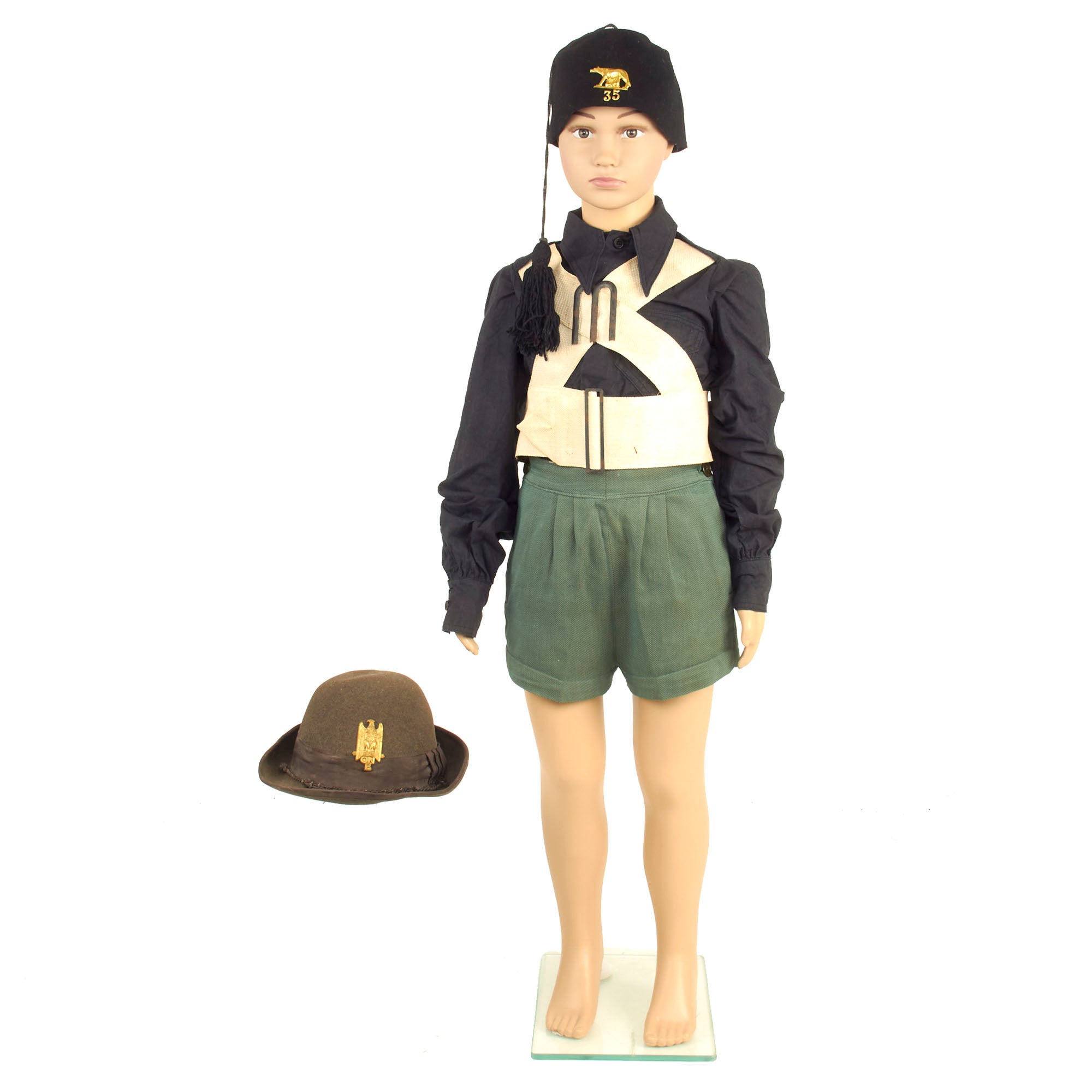The image is taken in portrait orientation and features a child-sized mannequin on the right, dressed in a distinctive outfit. The mannequin wears a black beanie-like hat with a long string and a big tassel. The beanie displays artwork of a creature, possibly a bear or leopard, along with the number 33 in orange. The mannequin is dressed in a black long-sleeved shirt and has a white strap crossing its chest, resembling a scout's uniform. It is also wearing green khaki shorts that reach just above the knees. To the left of the mannequin, there is a brown felt hat with a golden emblem, possibly an eagle, on a plain white background.